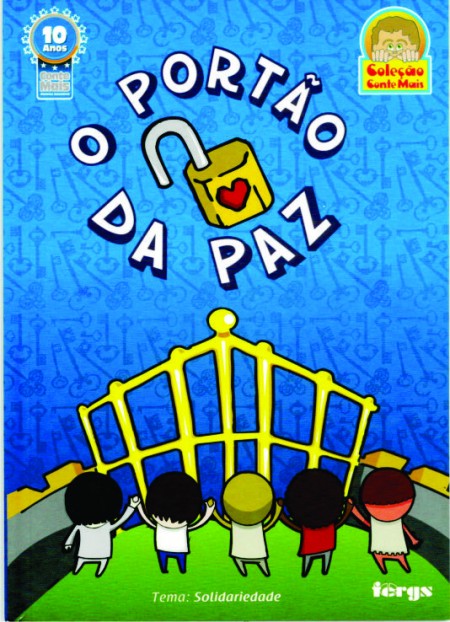The image depicts the cover of a book called "O Portal da Paz," characterized by a prominent light blue background adorned with various dark blue shadowed keys in a repeating pattern. Dominating the upper half of the cover is the book's title, "O Portal da Paz," written in bold white letters with blue borders, centered with an open padlock featuring a small red heart.

In the top left corner, there's a circular ribbon-like graphic with the white text "Ten Años" and below it, the words "Conte Más." The top right corner showcases a circle logo where a man peeks over a yellow rectangle, underscored by red text reading "Guilla Cal Gente Más."

Beneath the title, the illustration shows five children standing on green grass, holding hands with their arms raised. The children, shown from the back, are facing a large, ornate gold gate with a pyramid-shaped top, which has vertical bars and a cross member with a central ball. The background above the children is a gradient blue, lighter in the middle and darker toward the edges, enhancing the repeated key motif.

The overall design is a vivid and colorful photographic illustration, blending detailed graphics and text to convey a sense of peace and unity.